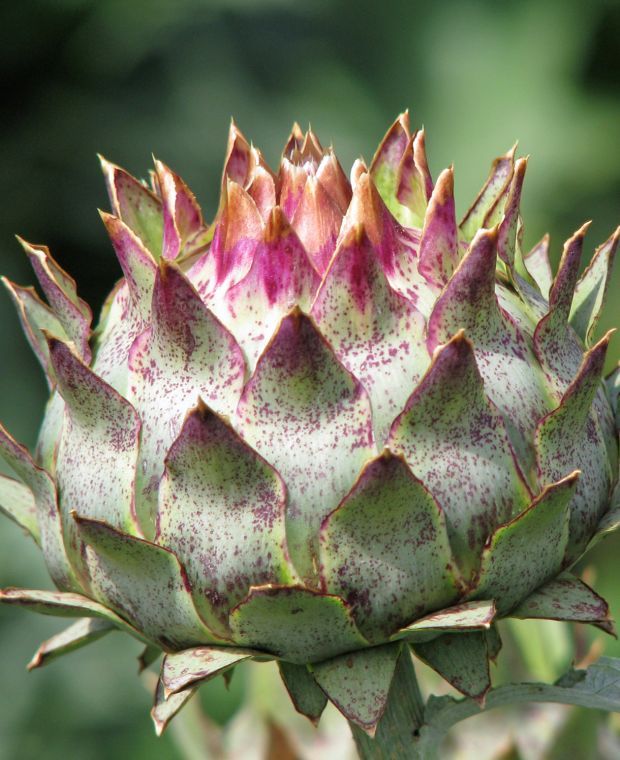This high-quality close-up photograph captures a unique plant that bears a striking resemblance to an artichoke, tulip, or even a dragon fruit. The plant features a bulbous, orb-shaped structure composed of several rows of pointy green petals with vibrant magenta pink tips, forming a beautiful gradient. The plant's round form is notable, becoming more pointed towards the center, and each petal is edged in a deep pink, contributing to its striking appearance. It rests atop a thick green stem, which also extends outward with a singular green leaf. The background of the image is artistically blurred, showcasing varying shades of green, gray, and black, which effectively highlights the plant's vivid colors and intricate details.